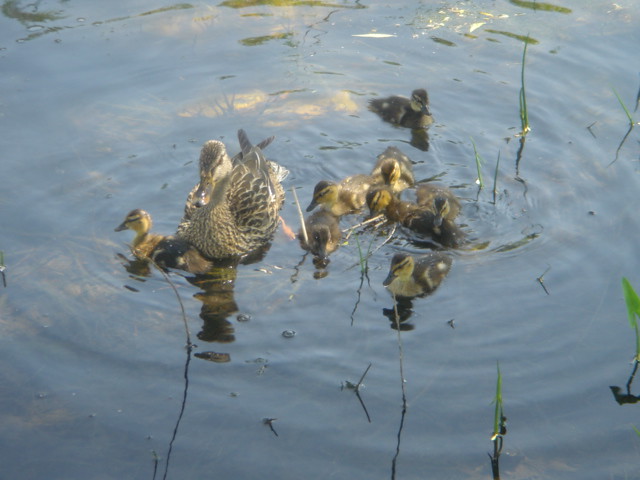In the detailed outdoor daytime photograph, we see a serene pond scene captured with slightly out-of-focus clarity. The image showcases a mother duck, prominently positioned left of center, guiding her eight ducklings as they swim. The mother duck, a mix of gray and brown with dark spots and an orange beak, faces a three-quarter view towards the lower left corner. Surrounding her, the ducklings, each with brownish heads, yellow chests, and light brown backs, frolic in the still water, creating gentle ripples. Most of the ducklings cluster to the right of their mother, while one ventures to her left in profile. The pond itself is tranquil, disturbed only by the movement of the ducks, with slight waves spreading from their playful activity. Green seagrass or weeds emerge from the lower right foreground, highlighting the natural setting. The good lighting of the scene casts a warm reflection on the water, adding to the overall calm and picturesque composition.